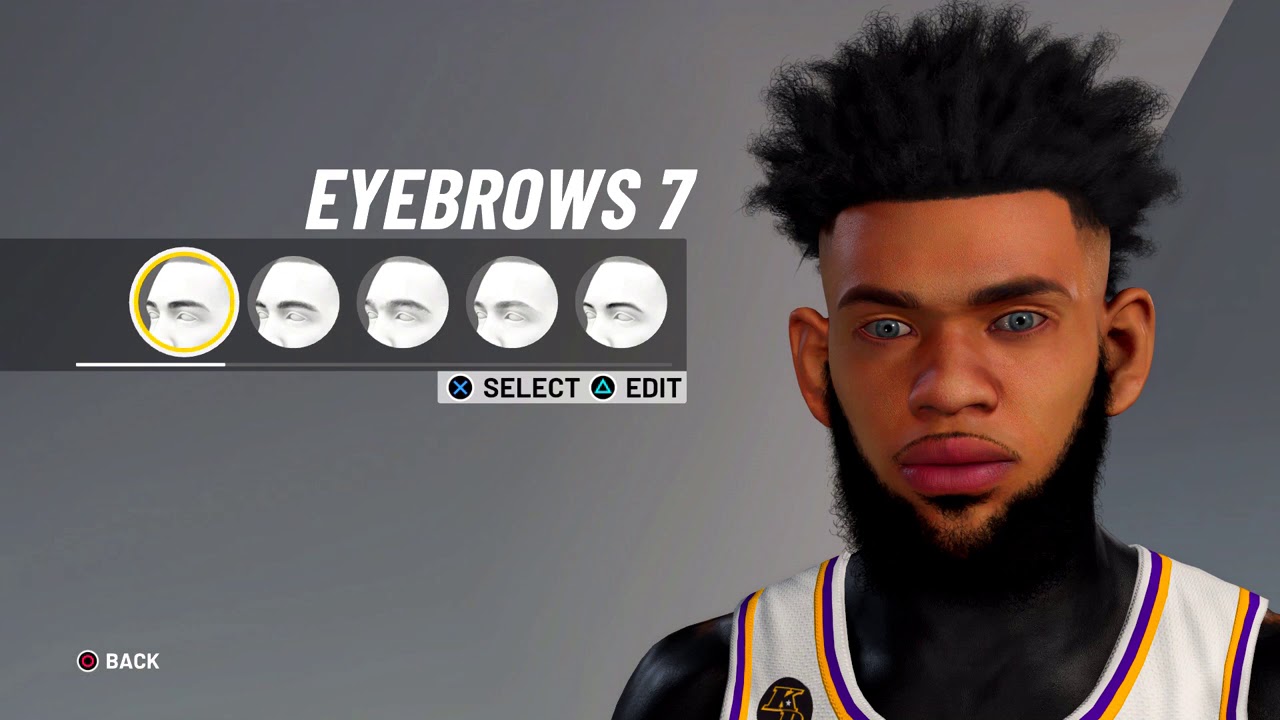The image is a detailed screenshot from a character customization interface in a digital sports game. The focus is on an African American male avatar, who appears to be modeled after a basketball player. This character has fluffy, curly hair styled upwards, a prominent square-shaped forehead, black eyebrows, and striking blue eyes. The avatar's facial features include a wide nose, a thin mustache just above his lips, a small goatee, and a connected full beard.

He is dressed in a visually striking jersey that features a blend of white, yellow, and blue colors, evocative of classic basketball team uniforms. To the left of the character, a section of the customization menu is visible, specifically focused on the eyebrows. It displays the label "Eyebrows 7" along with a row of five different eyebrow styles available for selection. The chosen style is highlighted as the first one on the far left. Additionally, navigation options such as "Select or Edit" and a back button are seen in the bottom left corner of the screen interface, indicating further customization features available to the user.